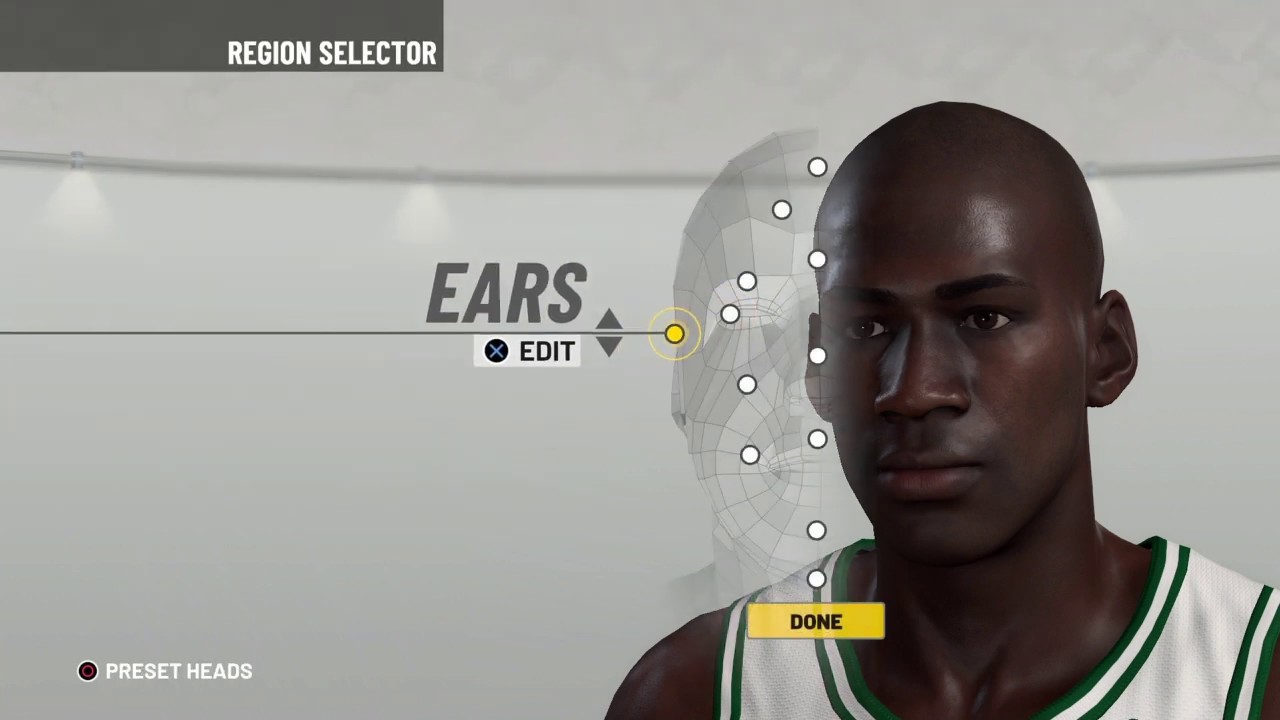The image depicts a detailed 3D model of a young African-American male, showcased within a character customization interface. He is dressed in a basketball-style sports jersey. The scene presents two versions of the model: the first is a fully realized 3D character, while the second is a skeletal, unfinished model featuring basic mesh lines, measurements, and editable parameters. 

The interface highlights various editable features including ears, eyes, eyebrows, forehead, mouth, nose, cheeks, chin, and neck, suggesting a highly customizable character creation system. A prompt indicating "Push X to edit" is visible next to the ears, illustrating interactive options for altering specific attributes. At the top left corner, a region selector is displayed, likely allowing users to choose different facial or body regions for detailed modifications. The current task appears to involve adjusting the character's ears. Overall, the image embodies a sophisticated character customization process, enabling extensive personalization for game avatars.